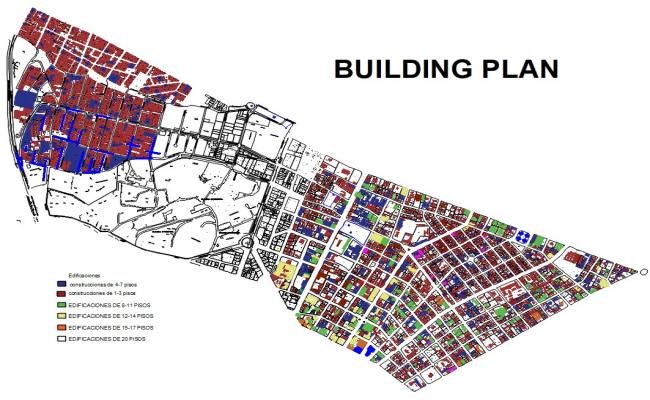The image displays a detailed, color-coded building plan of a city layout, presented from a bird's eye view in landscape orientation. The map occupies the central portion of the image, diagonally positioned from the top left to the lower right corner, resembling the shape of a bow tie. The urban design features a grid of streets intersecting various zones, designated by distinct colors including black, white, dark blue, maroon, green, yellow, orange, gray, and red with blue highlights. The upper right corner of the image prominently displays the bold text "BUILDING PLAN," while the bottom left corner contains a key with color codes, which are difficult to read due to their small font size. The map is a blend of illustration and cartography, with outlined sections indicating different areas for public gathering and business zones. The center section is predominantly black and white, transitioning to more colorful sections toward the edges. The overall presentation suggests that it may be a poster or sign, providing a comprehensive visual layout of the planned city.